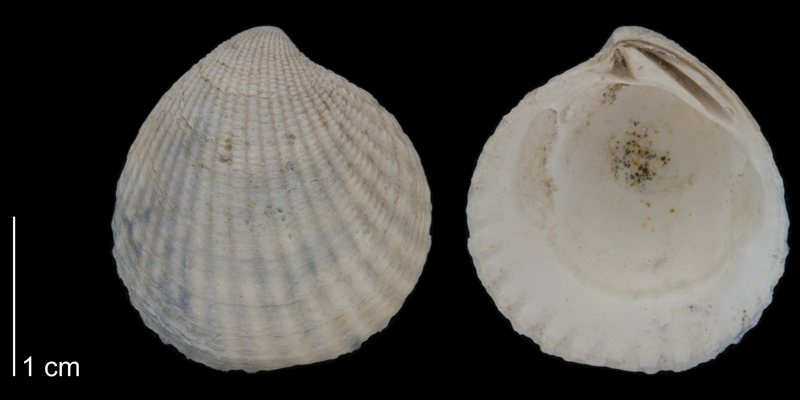This close-up color photograph features two seashells set against a deep black background, providing a stark contrast to their intricate details. The shells are positioned near the center of the image, slightly offset to the right. On the lower left side of the image, a white vertical line rises halfway up with the measurement "1 cm" beside it, offering a clear size reference.

The two seashells are displayed in different orientations, with the one on the left presenting its outer surface. This shell has a smaller, slightly pointy tip at the top, widening to a rounded base, and exhibits subtle texture and striations running from top to bottom with slight curvature. Its color palette includes shades of white, gray, brown, yellow, and occasional specks of orange.

The right shell shows the inner surface, smoother and paler compared to the outer shell. Notably, the interior has darker spots, which could be remnants of dirt. Both shells capture the essence of a natural collector's find, perhaps picked up from a beach, showcasing the varied textures and colors that characterize seashells.